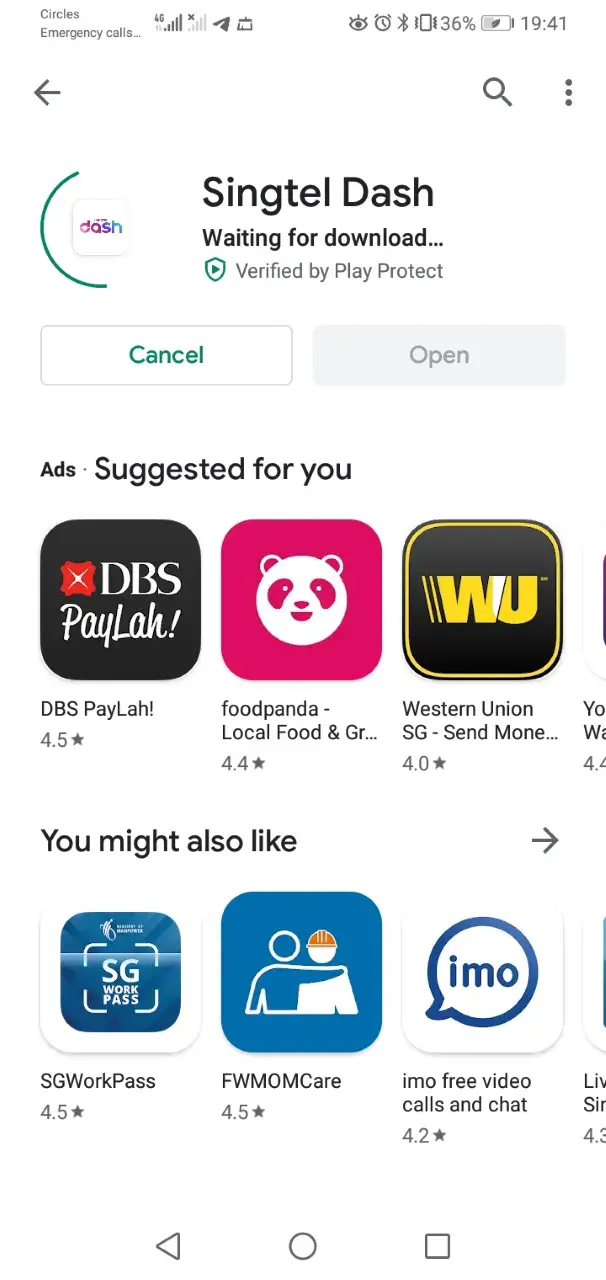The image is a smartphone screenshot of the Google Play Store, featuring the application "Singtel Dash" at the top of the screen. The app is in the process of being downloaded, as indicated by the text below its name, "Waiting for download..." Additionally, it mentions that the app is "Verified by Play Protect," ensuring its safety for download.

In the bottom section of the screen, there are two buttons: on the left, a "Cancel" button is visible, while on the right, a grayed-out "Open" button indicates that it is not yet available for interaction. The app's logo is displayed on the top left, with the word "Dash" where "D-A-S" is in purple and the "H" in blue, giving it a quirky, distinctive appearance. The download progress is visually represented by a green circle partially encompassing the logo.

At the top of the screen, the status bar shows it is 19:41 (7:41 PM), and the battery icon indicates it is almost halfway charged. This cohesive visual presentation suggests that the screenshot was captured from a smartphone.